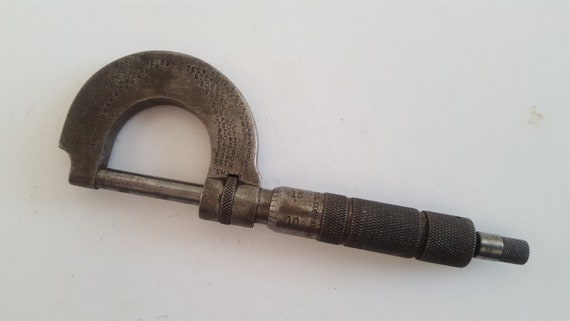The image showcases a metal tool, likely a wrench, prominently positioned against a white background. The tool, mostly silver with some brownish tones, displays significant signs of use and wear, marked with dark, greasy stains, particularly at its base and at the tip on the right side. The handle, characterized by its ridged texture, transitions from a smaller to a larger ridged section towards the top. The upper part features a thick, U-shaped hook with a metal rod extending towards the right. Despite the evident aging and greasiness, the tool's sturdy and heavy build is unmistakable.